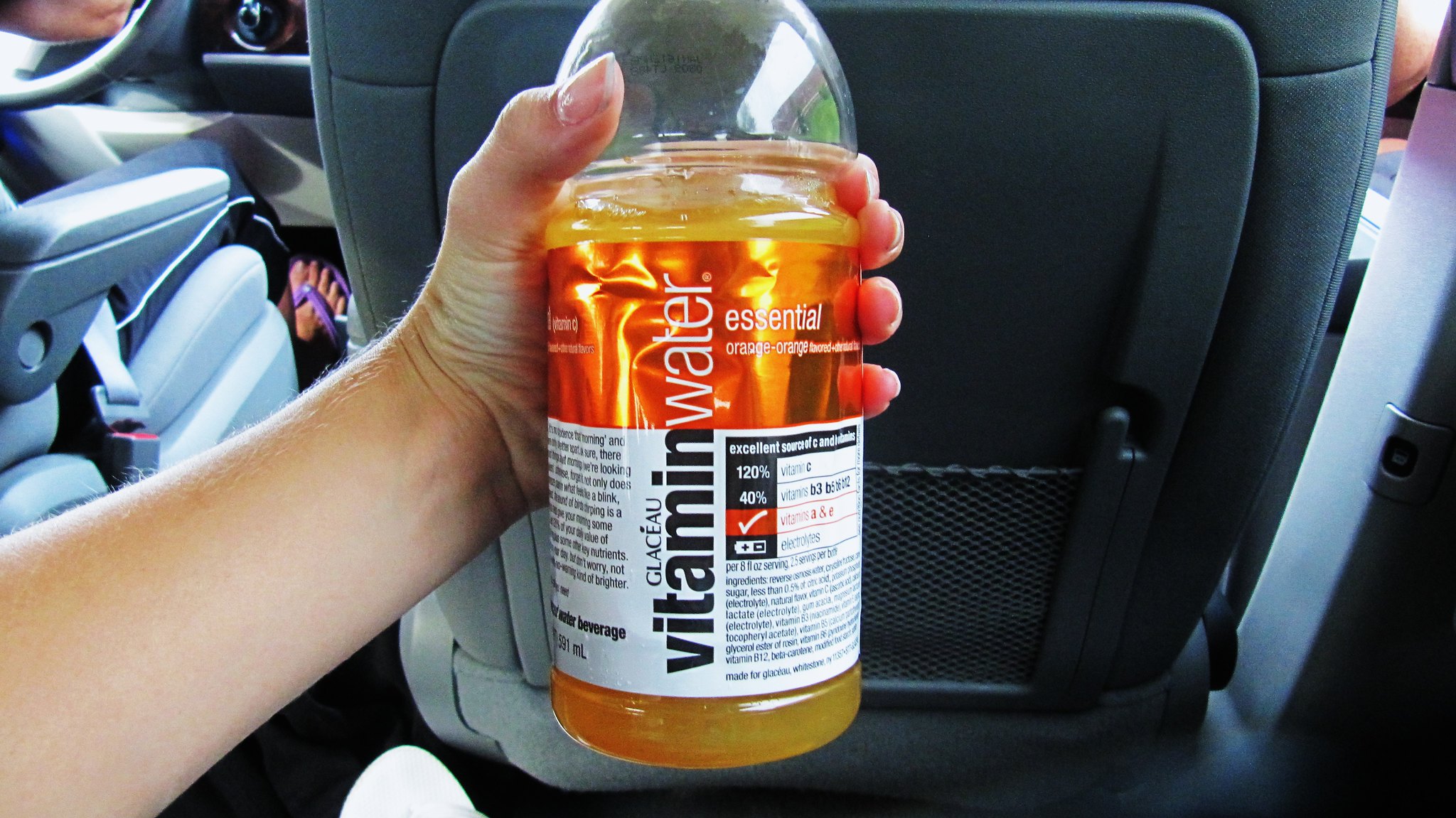This indoor color photograph captures a detailed scene inside a vehicle, likely taken from the backseat. Prominently in the center of the image, a left hand extends from the lower left, holding a partially full bottle of Glaceau Vitamin Water Essential. The clear plastic bottle contains an orange liquid. The label on the bottle features an upper goldish-orange section with the words "vitamin" in black and "water" in white, followed by "essential." Additional text on the label includes "orange, orange," nutritional percentages like "120%" and "40%," and a small red rectangle with a white checkmark, albeit partially obscured.

To the left in the upper corner of the photograph, the black steering wheel and the gray driver's seat are visible. The driver, another female, is identifiable by her purple flip-flop foot placed on the accelerator and a glimpse of her arm. The background consists of the gray backrest of the front passenger seat, reinforcing that the photo was taken from the backseat perspective. Overall, the photograph vividly juxtaposes the colorful labeled bottle against the muted interior of the vehicle.